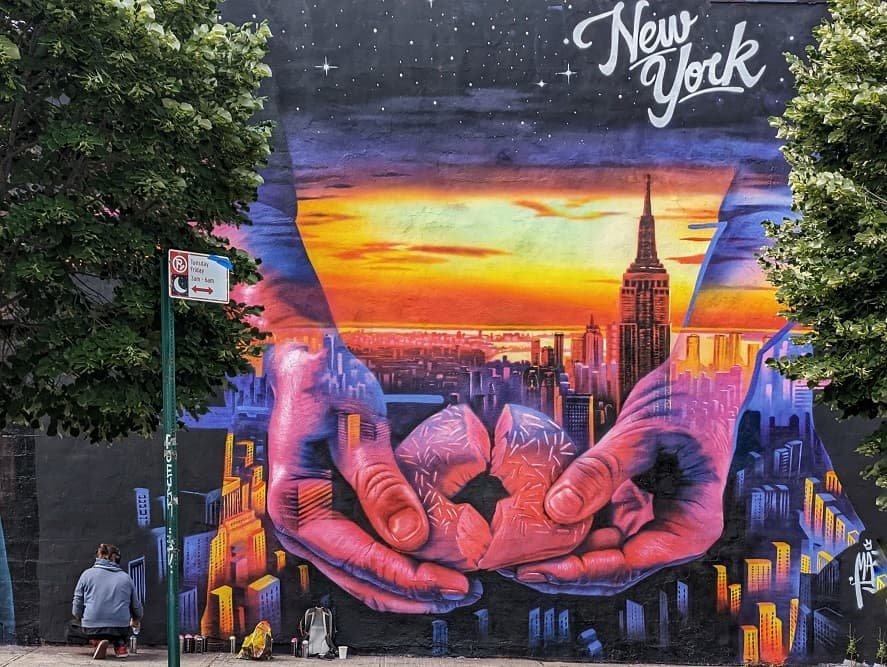The poster, designed as a mural on an exterior wall in New York, is a captivating composite of various elements. The central theme is the New York City skyline, prominently featuring the Empire State Building, beneath a dark sky scattered with stars. At the horizon, the colors blend into what appears to be either a sunset or a sunrise, suggesting a time of transition. The skyline is flanked by trees on both sides, adding a natural frame to the scene.

Dominating the upper portion are two hands descending from the sky, dramatically breaking apart a sprinkled donut, infusing the image with a surreal, almost religious sentiment. The words "New York" are elegantly scripted in white in the upper right corner. 

In the lower left, a solitary figure kneels, dressed in a blue hoodie with a backpack nearby, adding a human element to the otherwise celestial scene. A street sign or parking sign on a pole is also visible on the left side, grounding the mural in reality. The entire composition exudes a sense of mystique and wonder, blending the everyday with the extraordinary.